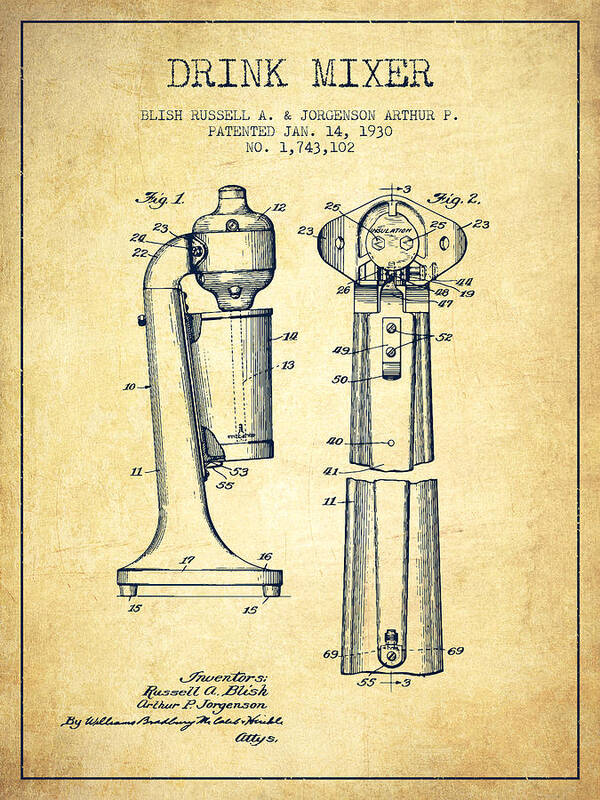The image depicts a detailed antique patent illustration of a drink mixer. The background has a paper-like, brownish light gray color, bordered by a black line forming a square. At the top, the faded lettering reads "Drink Mixer." Below this title, the names "Blish Russell A." and "Jorgensen Arthur P." are listed, along with the patent date, "January 14, 1930," and the patent number "1,743,102." The illustration showcases two views of the mixer: a side view and a rear view. Both views feature detailed labeling of the various parts with numerous numerical identifiers. The apparatus itself includes a bulb-like top, angled at 90 degrees to the left, with a cup in the middle. In the bottom right corner, the inventors' names, "Russell A. Bliss" and "Arthur P. Jorgensen," appear alongside the name "William Bradley" and the term "attorneys." The drawing is meticulous, identifying every component, down to the screws and bolts, although no key is provided to explain the numbered parts.